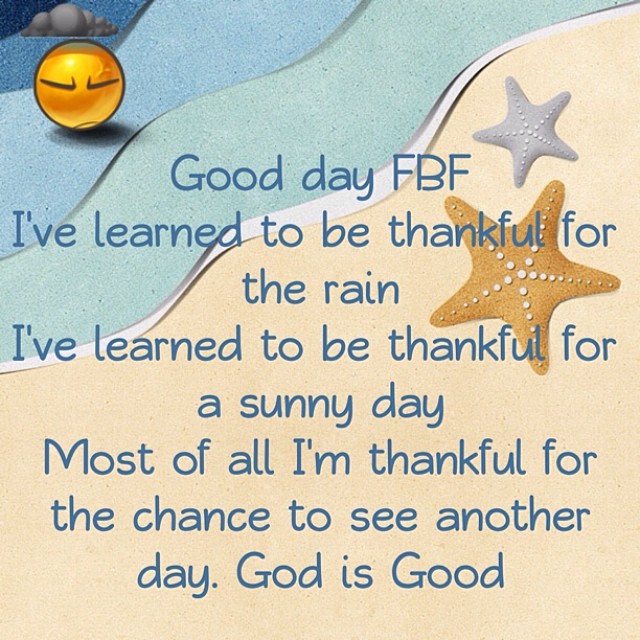This color image, widely recognized as a meme on social media, features a digitally illustrated beach scene, composed of shades of blue and green symbolizing water, with hints of white and beige for the sand. On the right side of the image are two starfish, one gold and one silver. In the top left corner, there is an emoji with a sad face under a storm cloud, emphasizing a mix of emotions. The text, written in a blue comic-style font, reads: "Good day FBF, I've learned to be thankful for the rain. I've learned to be thankful for a sunny day. Most of all, I’m thankful for the chance to see another day. God is good." The entire image has a graphic, cartoony look, with separations between each color resembling a paper cut-out style.